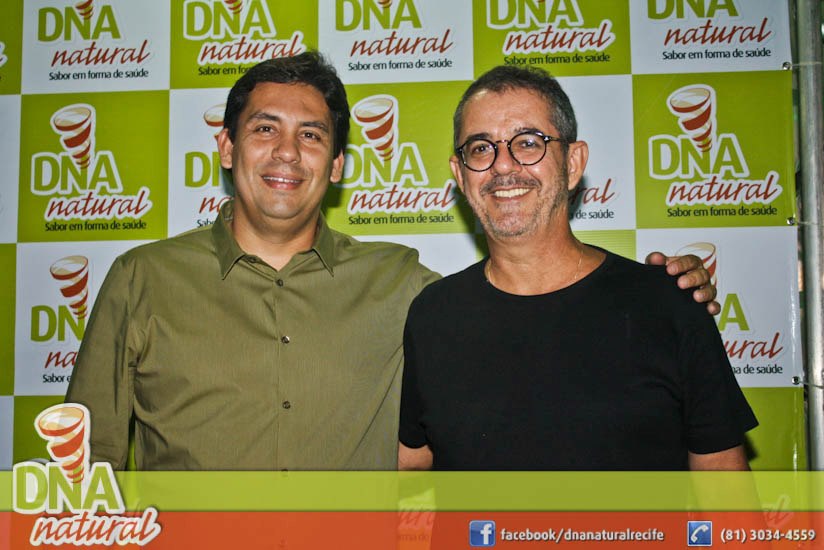In the photograph, two middle-aged men are smiling at the camera. The man on the left, dressed in an olive-colored button-up shirt with black buttons, has his hand placed on the shoulder of the man beside him. The man on the right is wearing a black t-shirt and sporting black round-framed glasses, a mustache, and some stubble. Both of them are smiling warmly. They are standing in front of a checkered poster featuring alternating green and white squares. The poster, which seems to be canvas material secured with zip ties to a metal pole visible at the right edge, prominently displays the text "DNA Natural" written in green capital letters, with the word "Natural" in red cursive beneath each "DNA." There is more text in black, but it's not fully legible. At the bottom of the poster, an additional strip includes the "DNA Natural" branding alongside a green and orange stripe, with Facebook and contact information. The overall setup suggests they are posing at an event or promotional backdrop.